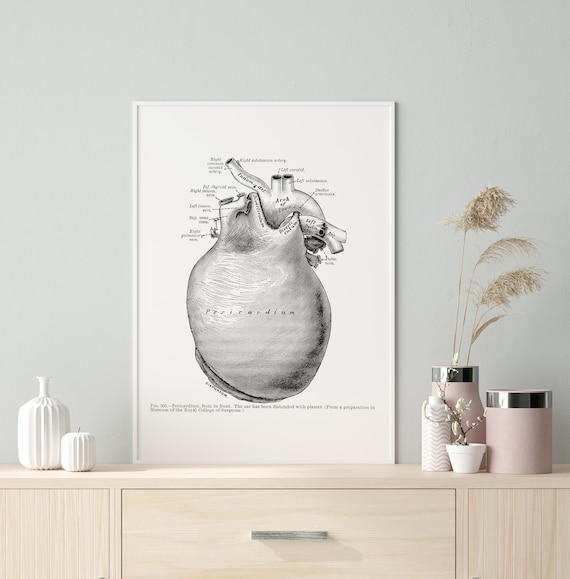In this detailed image, the setting appears to be a minimalist room or office, featuring a light-colored wooden dresser that serves as a central piece of furniture. Positioned on the dresser is a black-and-white poster showcasing an intricate pencil sketch diagram of the heart, prominently labeled with terms such as "pericardium" among others, though the small and unclear writing makes it difficult to discern all the labels. 

The dresser is adorned with several decorative items: on the left side, there's a white pot and a white candle, while on the right, there are two light pink containers. One of these pink containers has a faux plant resembling wheat or hay sprouting from it, adding a natural touch to the setting. Additionally, there's a small potted plant in a white vase with green leaves, subtly contributing to the room’s decor.

The entire scene is set against a white wall, creating a stark, simple background that accentuates the detailed anatomical poster and the carefully arranged decor items. The metal handles on the dresser add a touch of modernity and functionality to the overall aesthetic of the space.